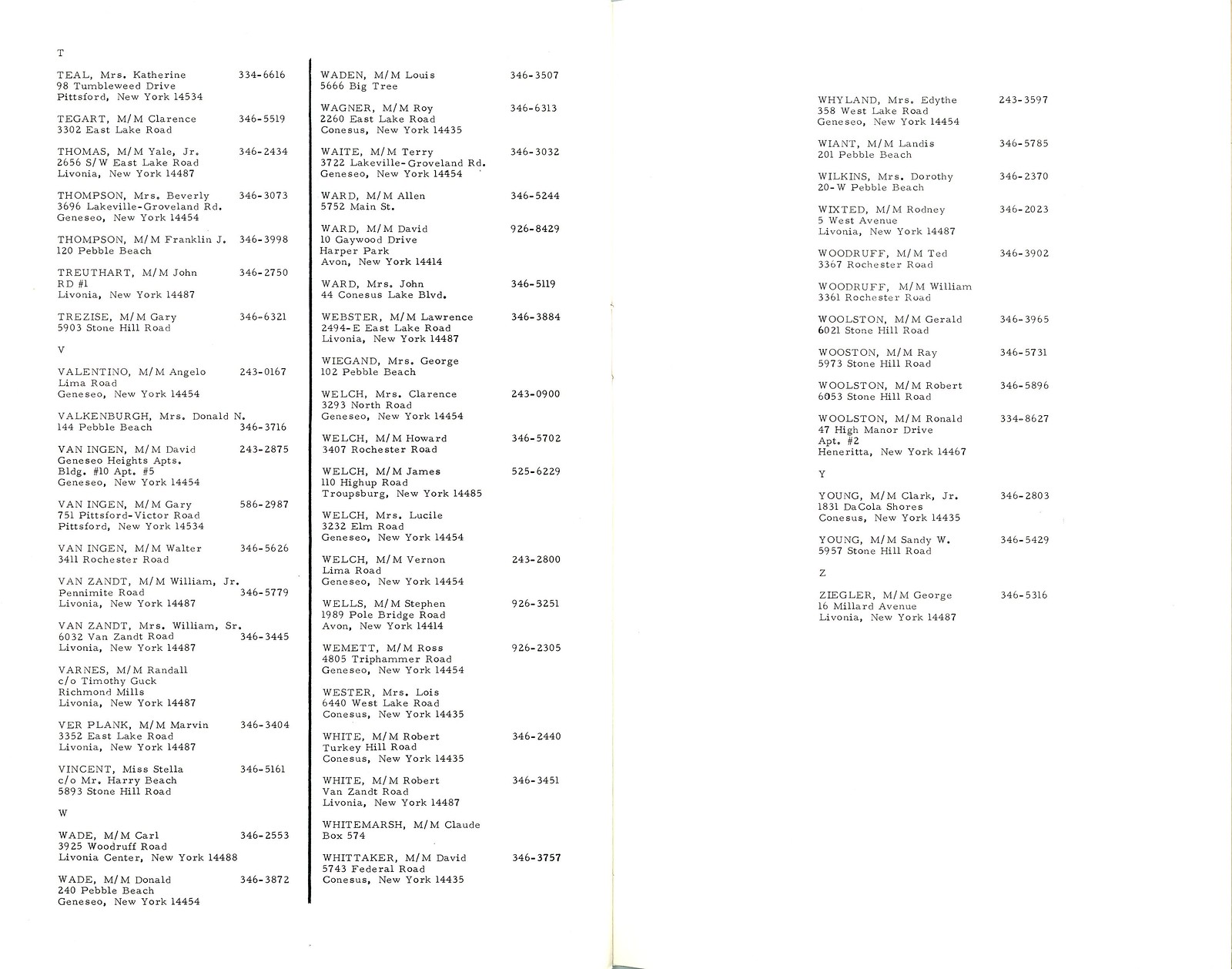The image appears to be a scanned page from a phone book, featuring a detailed list of names, addresses, and phone numbers organized into three vertical columns. The entries are alphabetically arranged by last names. For instance, one entry in the "T" section reads: "Teal, Mrs. Catherine, 98 Tumblewood Drive, Pittsford, New York, 14534," followed by the phone number "334-6616." The page shows various localities, including Livonia, Pittsford, Geneseo, Avon, and Henrietta within Monroe County. The columns on the left side of the page are separated by a vertical black line, while a single column exists on the far right. The background features a light yellow line running down the middle of the page, further dividing the sections. The page also includes a smaller number of entries in the "Y" and "Z" sections, with only two names under "Y" and one under "Z."